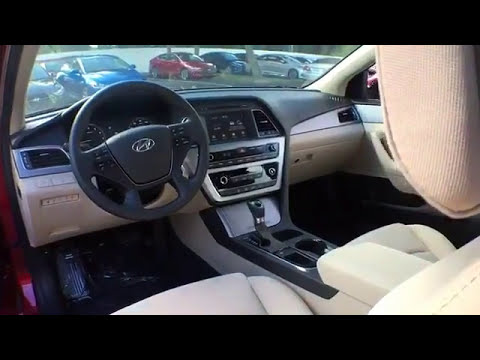The image portrays the interior of a brand-new Hyundai vehicle, as suggested by the visible Hyundai logo on the center of the black steering wheel. The view is from the driver’s side door towards the dashboard and steering column. The vehicle's seats and inner door panels are upholstered in light tan fabric, possibly corduroy. The interior features a black dashboard adorned with silver trim underlining the edges and surrounding the center controls, which include a radio, temperature dials, and a touchscreen display. The center console, equipped with a shifter and cup holders, is predominantly black, with the armrest section in a cream color. The floorboards are covered in protective plastic, hinting at the car's newness. The dashboard also contains a total of four air vents, two positioned for the driver and two for the passenger. Both the glove compartment and the area beneath the dashboard are cream-colored. Through the windshield, a parking area is visible, populated with several cars, indicating that this might be a car dealership or a parking garage. The vehicles visible outside are of varying colors, including white, blue, red, and black.